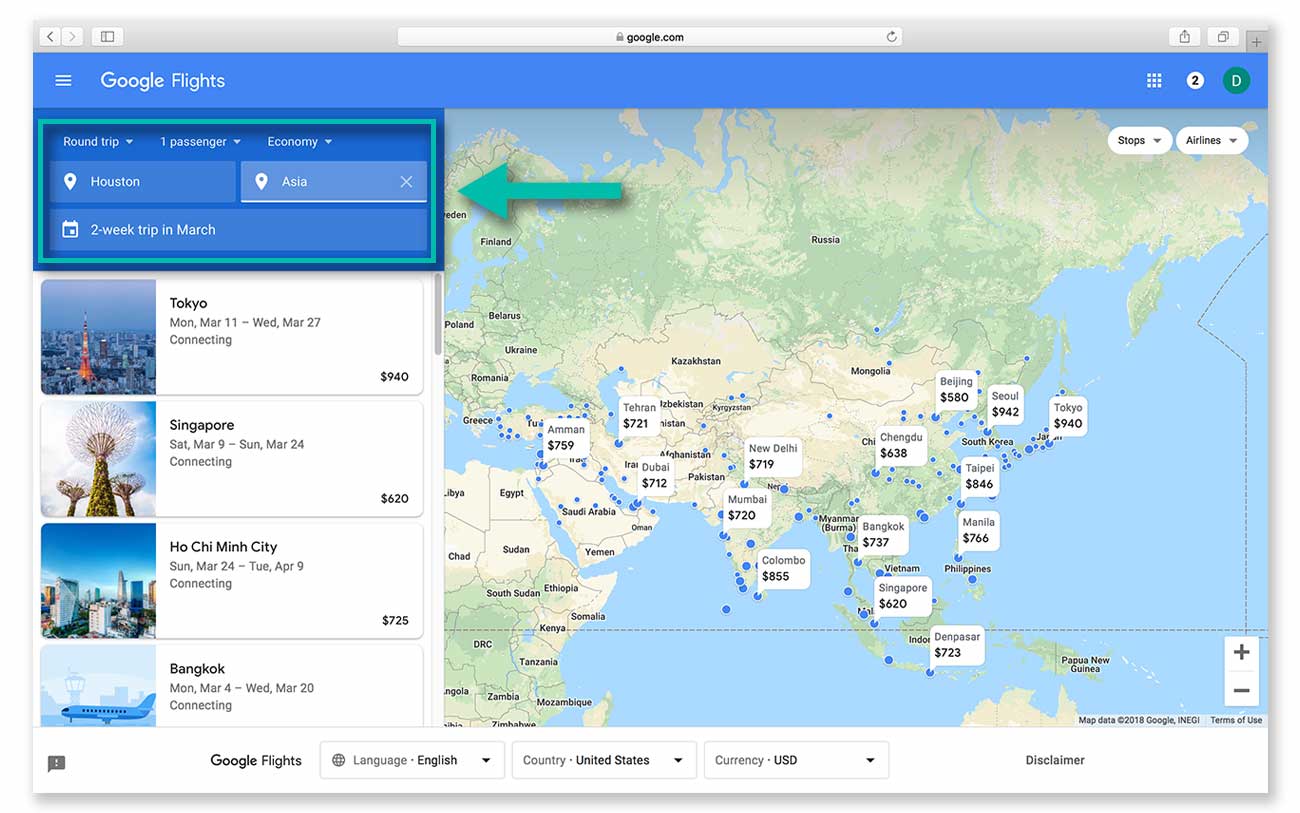A rectangular screenshot captures the interface of the Google Flights website. The top portion of the image features the Google Flights logo in white text, set against a dark blue background that serves as a border. Below this header, a highlighted blue section with a teal outline is prominently displayed. A large green arrow points to this blue section, indicating where users input their flight details.

In the designated fields, the origin is clearly marked as "Houston" and the destination as "Austin," both written in white letters. Beneath these fields, a white background showcases a list of suggested tourist destinations in black text. The first destination listed is Tokyo, followed by Singapore, Ho Chi Minh City, and Bangkok. Each destination is accompanied by an image to its left.

On the right side of the screenshot, a large map features prominently, depicting regions of Asia and Africa. The map uses a color scheme of whites and greens, denoting forested areas, with blue hues representing oceans and other bodies of water.